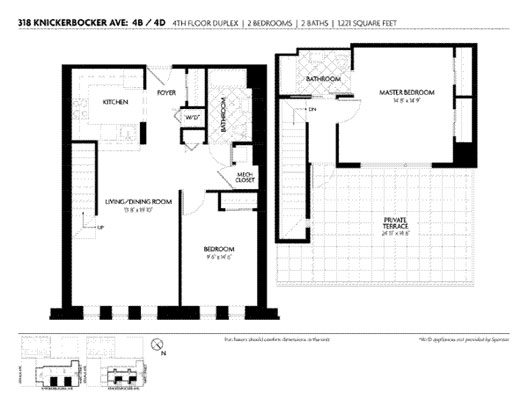This detailed architectural drawing depicts a fourth-floor duplex apartment located at 318 Knickerbocker Avenue, units 4B and 4D. The black and white blueprint outlines a spacious two-bedroom, two-bathroom layout encompassing 1,221 square feet. The duplex has two distinct sections, presumably side-by-side units, as indicated by their respective labels.

In the second unit, which appears more detailed in the drawing, the layout features a master bedroom complete with a private terrace, a substantial closet, and an en-suite bathroom. Adjacent to this master suite is a smaller bedroom with its own closet. Additionally, there is an extra large closet in the hallway and another spacious bathroom. The common areas include a fully-equipped kitchen and a combined living and dining room space, promoting an open-concept design. A stairway is noted, indicating access to the master bedroom situated on an upper level.

The blueprint also includes a smaller inset drawing, presumably of a related structure showing a two-car garage attached to a compact house, though its exact purpose remains unclear. The apartment’s entrance is conveniently located off the kitchen, nestled between the kitchen area and the first-floor bathroom, enhancing ease of access and flow within the home.